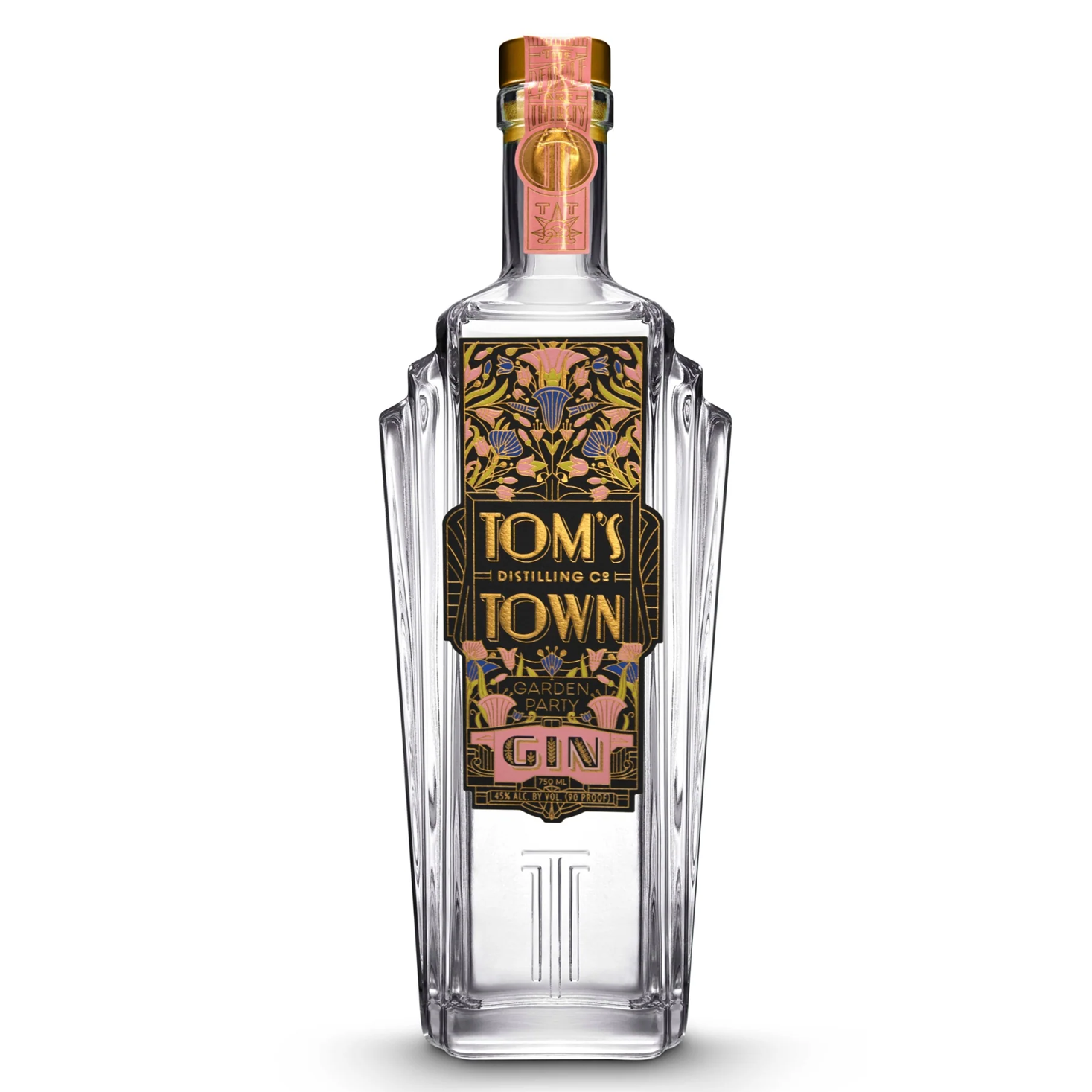This color photograph features a clear glass bottle of Tom's Town Gin, set against a plain white background. The bottle is sealed with a brown cap adorned with a pink seal, which has gold print on it. The front of the bottle showcases an intricate label with a kaleidoscope design, combining stylized flowers and leaves in pink and blue on a black background, giving it a visually striking effect. A black band across the middle of the label prominently features the text "Tom's Town" in large gold letters, with "Distilling Company" in smaller print between the words. Towards the bottom of the label, in the pink section, "Garden Party" is displayed, with "Gin" written in small, decipherable print beneath it. The overall effect is a highly decorative and visually appealing bottle that effectively advertises the brand’s unique aesthetic.